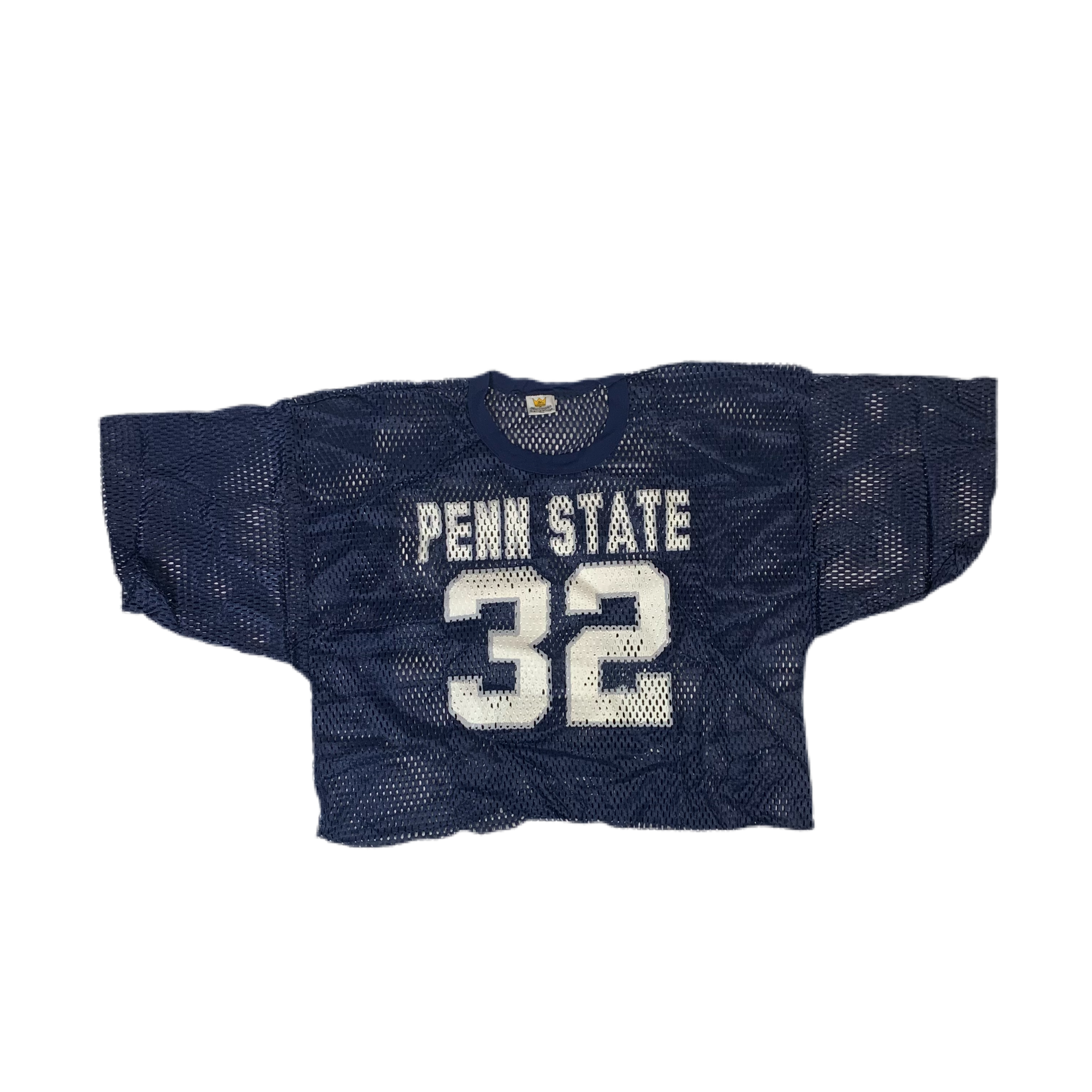In this image, we see a dark blue mesh football jersey, prominently featuring a Penn State design. The jersey is made from a fishnet material, making it very see-through with numerous holes scattered throughout, providing a highly breathable feel. It lies flat against a plain, white background, showing only the upper portion from the mid-stomach upwards, where the arm areas are flattened to the sides. This short-sleeved, crop top-styled jersey is not intended for professional play but more for training or casual wear, exposing the lower half of the stomach when worn. Across the center of the jersey, the words "Penn State" are displayed in large, white, uppercase letters, and directly below, the number "32" is prominently printed in white. Interestingly, the perforations typical of the mesh material are inconsistently applied to the numbers, with some parts remaining solid white.